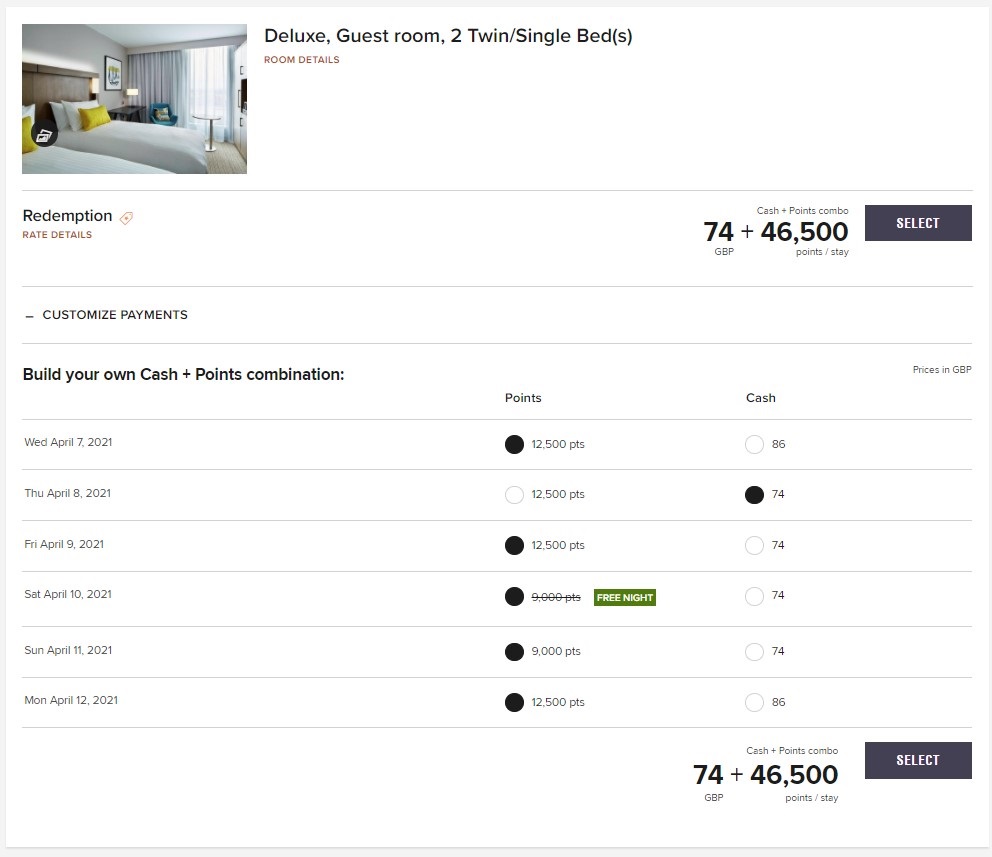The checkout page of the website displays a hotel room booking interface set against a clean, white background. In the upper left corner, there is a sample image of the deluxe guest room, which boasts two twin beds adorned with white comforters. Each bed has a stack of three pillows: two white and one small yellow. The room's decor includes a brown headboard with an overhead light, a framed picture on the wall, a solitary black desk accompanied by a lamp, a blue chair next to a small round table, and curtains drawn halfway, allowing natural light to float into the room. 

Directly beneath the image, the text "Deluxe Guest Room, Two Twin-Single Bed(s)" followed by "Room Details" in orange is displayed. A light gray dividing line separates this section from the next. Below it, the "Redemption" section includes an orange tag icon and the text "Rate Details" in orange, with the cost listed as "74 GBP plus 46,500 points - Stay." Above that, the text "Cash plus Points Combo" is highlighted, and a black button labeled "SELECT" in white capital letters stands out to the right. 

Further down, another dividing line appears, leading to the "Customize Payments" section, followed by a list for building your own cash and points combination. To the far right, prices are noted in GBP, with separate columns for points and cash. 

Each row reflects daily options:
- Wednesday, April 7th, 2021: 12,500 points selected, 86 GBP not selected.
- Thursday, April 8th, 2021: 12,500 points not selected, 74 GBP selected.
- Friday, April 9th, 2021: 12,500 points selected, 74 GBP not selected.
- Saturday, April 10th, 2021: 9,000 points selected with a strikethrough, indicating a free night in a green box with white text. 74 GBP not selected.
- Sunday, April 11th, 2021: 9,000 points selected, 74 GBP not selected.
- Monday, April 12th, 2021: 12,500 points selected, 86 GBP not selected.

At the bottom, "74 GBP plus 46,500 points - Stay" is reiterated, with "Cash and Points Combo" above it and another black "SELECT" button to the right, featuring white text in capital letters.